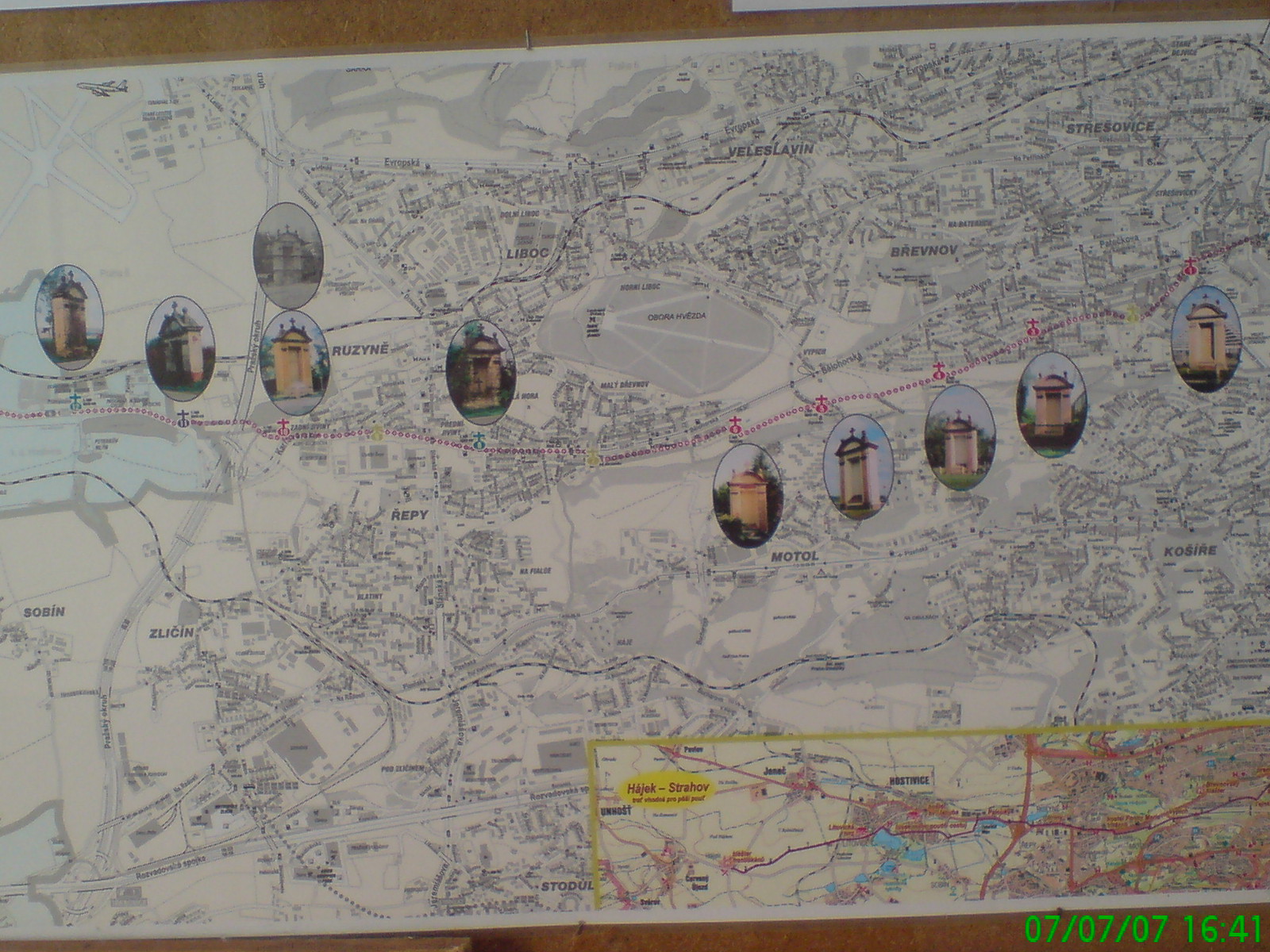This image depicts a detailed map with a predominantly white, gray, and black color scheme, accentuated by various colored highlights. The map features a brownish background at the top and bottom portions. Numerous red markings, including a prominent dotted red line, traverse the map. Scattered across the map are small oval windows containing images of what appear to be different buildings or perhaps crypts and mausoleum entrances, all sharing a similar shape. 

A significant section near the bottom right is distinctively colored with light yellow, red, blue, and green accents. Amidst this section, a yellow rectangle contains lines primarily in light red along with a blue and yellow shape bearing red text too small to decipher. Additionally, light blue representations of bodies of water are visible on the left side of the map.

The locations and text on the map are in an unidentified language, adding a layer of mystery to its origin. In the bottom right-hand corner, the neon green text reads "07/07/07 16:41," indicating a date and time.